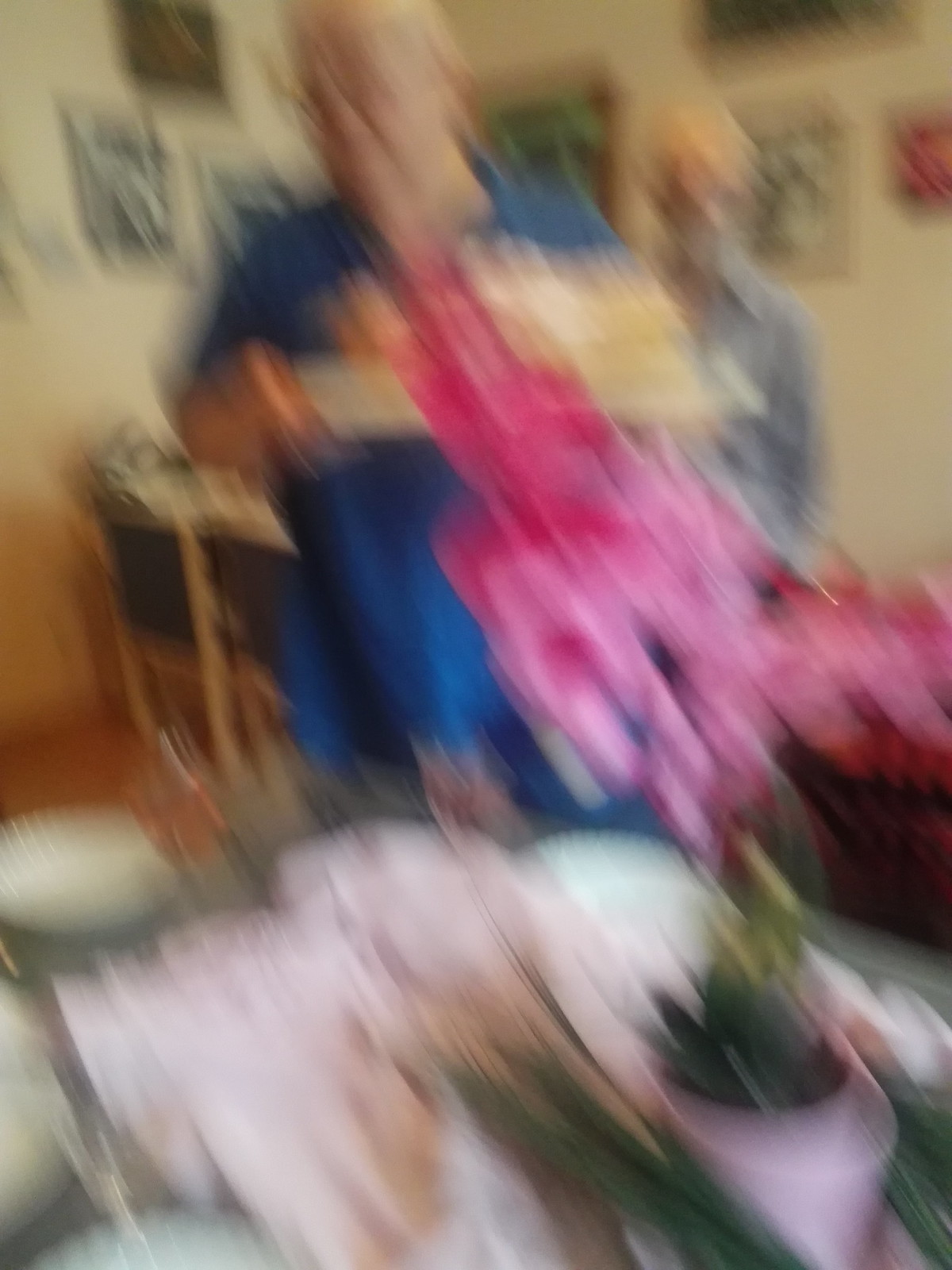A very blurry photo captures a scene with two people standing at a table, suggesting the setting might be a celebratory event, possibly a birthday party. The person closer to the table appears to be holding a platter, which might be a birthday cake. The table in the foreground is adorned with decor, including an orchid in a pot, numerous plates, and green linens. Behind the two individuals, there is a second similarly set-up table. The walls are decorated with various pictures, adding to the festive or restaurant-like ambiance. The overall impression is that the photo was taken hastily, adding to its blurred condition.